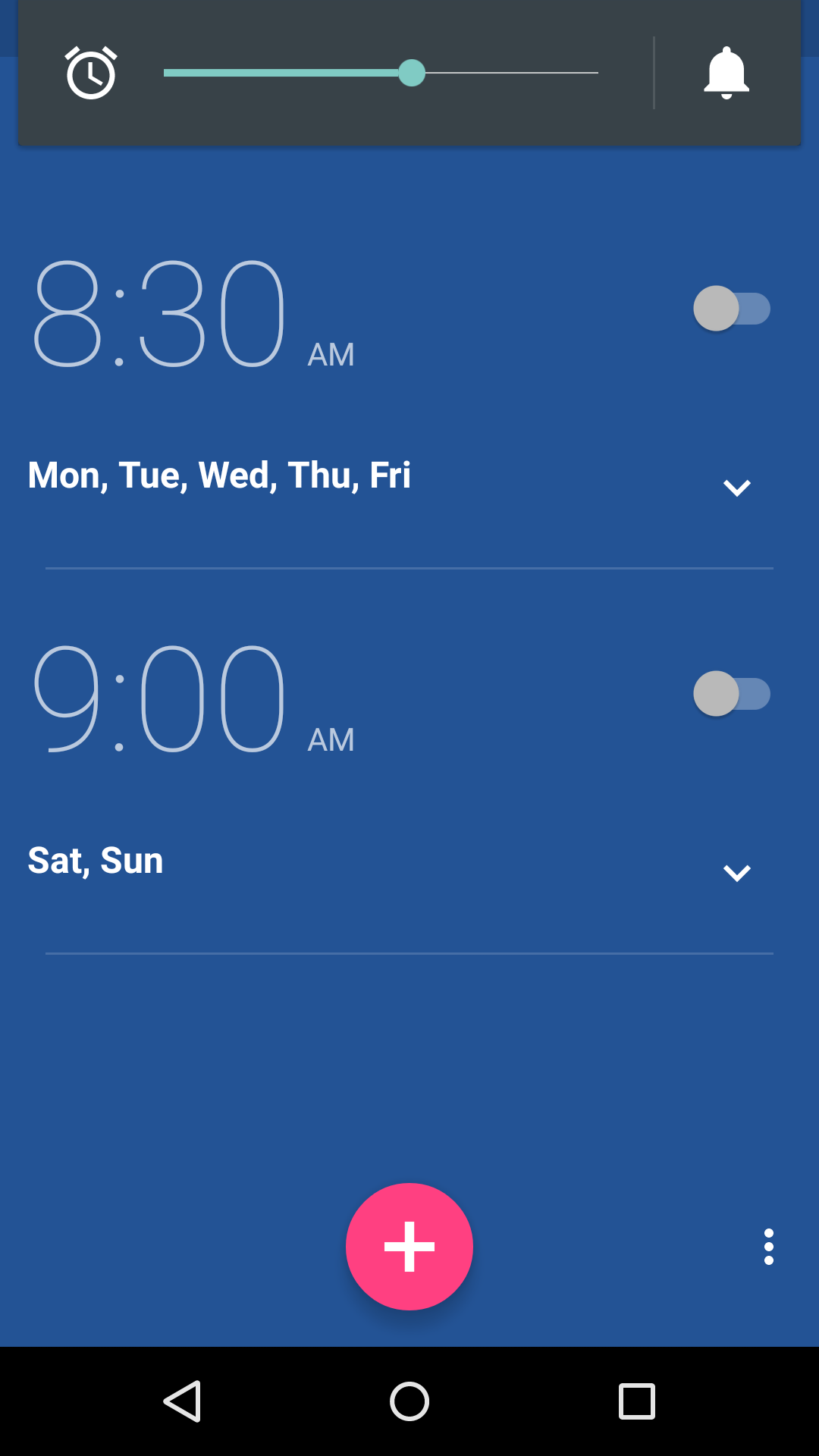This is a screenshot taken from a smartphone displaying the alarm clock settings. The background is navy blue with white text. At the top, there is an alarm set for 8:30 a.m. with a gray toggle switch in the left "off" position. Beneath this, in bolder white text, the days of the week for this alarm are listed as "Mon, Tue, Wed, Thu, Fri," indicating workdays, accompanied by a downward arrow to the right.

Below that, there is a second alarm set for 9:00 a.m., also with a gray toggle switch in the left "off" position. The days for this alarm are abbreviated as "Sat, Sun," representing the weekend, with another downward arrow to the right.

At the bottom of the screen, there is a white plus sign within a pinkish-red circle, which likely serves as a button to add a new alarm. The very bottom of the screen features navigational icons in a black rectangle: a triangle, circle, and square from left to right.